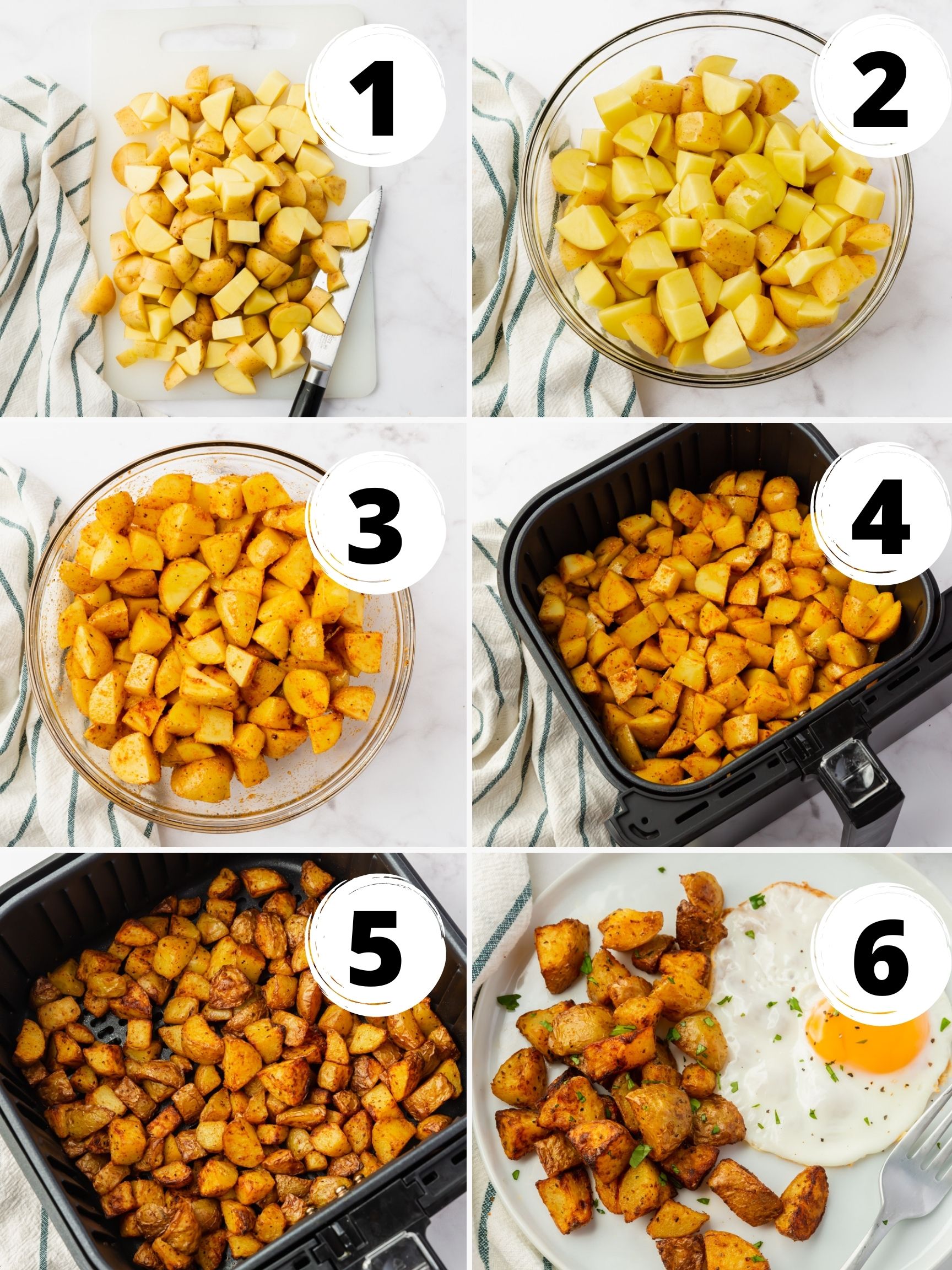This full-color, staged indoor image consists of a six-part step-by-step guide labeled 1 through 6, showing the process of making air-fried potatoes. Each of the six numbered squares is arranged in two columns and three rows. In the top left image (1), there is a silver knife with a black handle on a cutting board amid cubed potatoes, adjacent to a white napkin with green stripes. The top right image (2) displays these cubed potatoes in a clear glass bowl. The image to the left in the middle row (3) shows the same bowl of potatoes, now seasoned, hinting at a darker hue. Moving to the image to the right in the middle (4), the seasoned potatoes are placed inside the black, square tray of an air fryer, which is visibly deep with a handle extending downward. The bottom left image (5) showcases the cooked potatoes in the air fryer tray. Finally, the bottom right image (6) presents the finished dish: the crispy, golden air-fried potatoes served on a white plate with a sunny-side-up egg garnished with green parsley, accompanied by a silver fork. The continuity of the white napkin with green stripes appears subtly in the background of each stage.